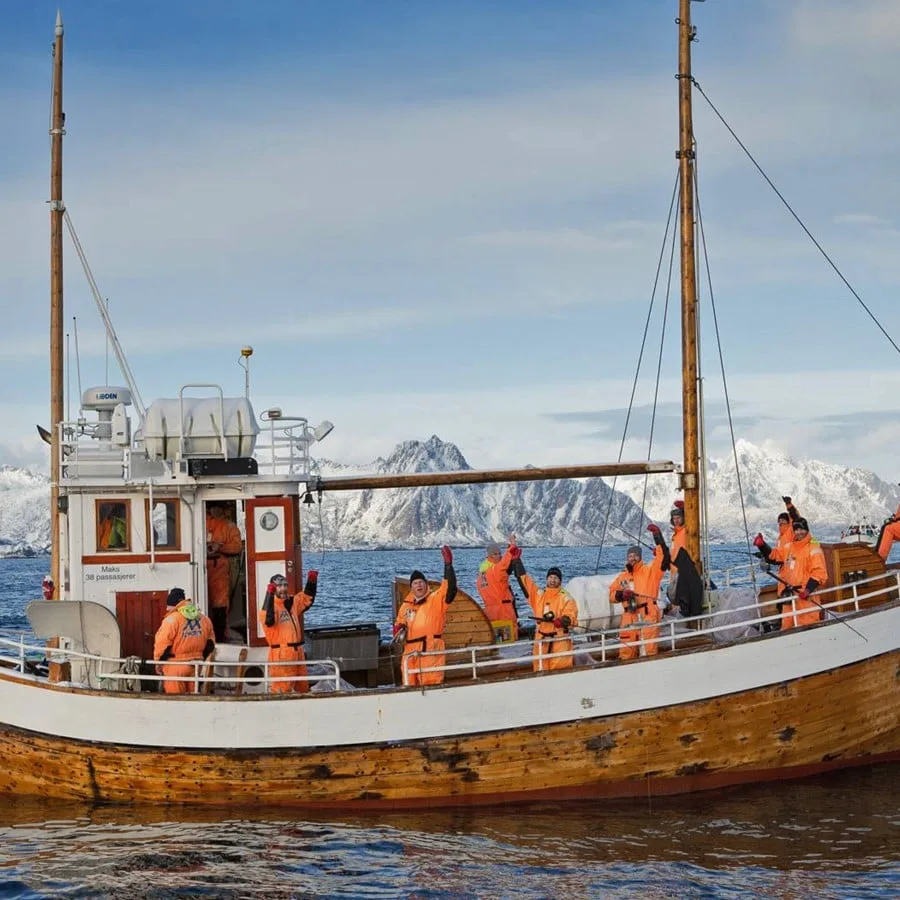This striking photograph features a wooden sailing boat, adorned with a white trim and a silver railing, set against the breathtaking backdrop of a tranquil Antarctic or Arctic seascape. The serene blue sky occupies the top half of the image, lending a vivid contrast to the towering, snow-capped mountains and icebergs that dominate the horizon.

The boat, which stretches across the frame from left to right, is populated by seven men clad in heavy orange jackets and jumpsuits, likely due to the frigid conditions. Some men face the camera while others look away, with several raising their arms in what seems to be a gesture of triumph or greeting. The second man from the right has both arms aloft, mirrored slightly by the adjacent men who also raise their hands.

Prominently situated on the deck is the captain's quarters, a red and white structure directly facing the camera, complete with a visible luggage storage compartment on top. Despite the absence of sails, the vessel sports two brown beams with wires, indicating its potential as a sailing ship. The water beneath the boat appears somewhat murky, reflecting the chill and ambiguity of the surrounding icy expanse. The overall scene beautifully captures a moment of human endeavor against the stark, icy majesty of the polar region.